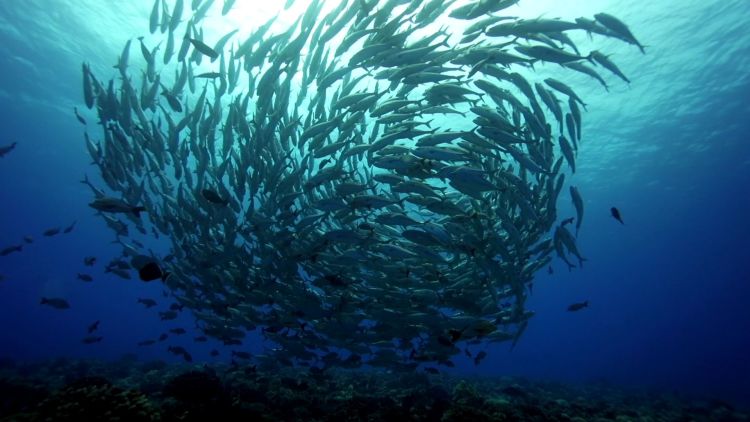This detailed underwater photograph captures a stunning scene where hundreds of fish form a giant swirling mass, resembling a whirlpool or cyclone. The swirling school of fish is positioned in the center of the image, with several of them scattered on the sides. The fish display various sizes and some possess a silvery sheen, though specific details about their species are indistinguishable. The vibrant gradient of the water ranges from bright aqua at the surface, where the sunlight penetrates, to darker shades of blue and eventually purple as the depth increases. At the very bottom, a hint of the ocean floor is visible, dotted with green plants. The overall effect is an ethereal underwater landscape, with the central swirl of fish standing out dramatically against the gradient backdrop.